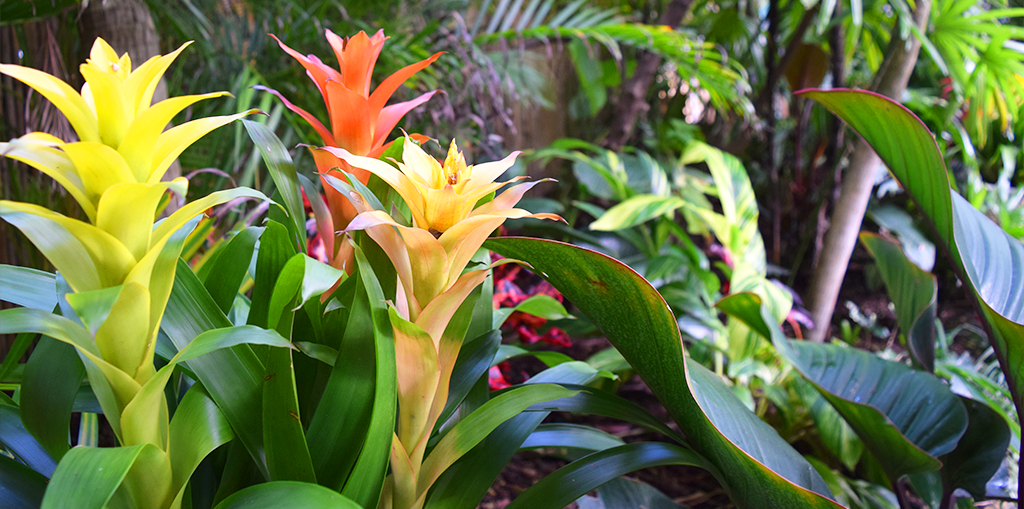This detailed and vibrant photograph captures a striking array of tropical flora, showcasing a high-contrast scene filled with lush plants and colorful flowers. In the foreground, three prominent flowers catch the viewer's eye: a bright highlighter-yellow bloom on the left, an orange blossom slightly recessed in the center, and a lighter yellow flower on the right. These flowers are surrounded by thick green leaves, with the right side featuring particularly large, elephant ear-like leaves that add to the foliage's grandeur.

Further enhancing the composition, the background, though slightly out of focus, reveals a tree trunk and an array of smaller red and purple flowers, creating depth and a sense of a rich, layered tropical environment. The vibrant greens, along with the different shades of yellow, orange, and touches of red, dominate the color palette, giving the scene a lively and exotic feel, reminiscent of a Hawaiian or similarly tropical locale. The photograph appears to be taken during the day, showcasing the plants and flowers basking in the sunlight, which highlights their vivid colors and intricate details. Overall, it is a striking and professional-grade image that beautifully captures the essence of tropical beauty.